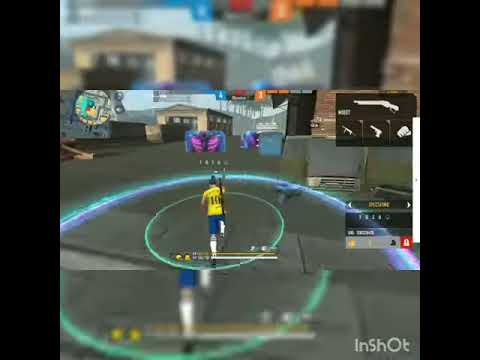The image is a screenshot from a video game, prominently displaying an in-shot watermark text "InShot" in the bottom right corner. Vertically oriented black strips frame both sides of the image. Central to the scene, an avatar wearing a yellow jersey with the number 10 and blue shorts is positioned. He is encircled by a green glowing ring, and a larger, turquoise semi-arc surrounds this circle. The character appears to be holding a weapon, perhaps a gun, while standing on a dark gray surface. The background features a beige building partly obscured by a purple-magenta object resembling lungs. The upper right corner of the image includes a display menu showcasing various weapons, including a shotgun, machine gun, handgun, and a fist icon. Adjacent to this, there is another display with indistinguishable text and two sided arrows. Additionally, the upper left corner features a map with a highlighted area, indicating the avatar's position within the game's urban environment.